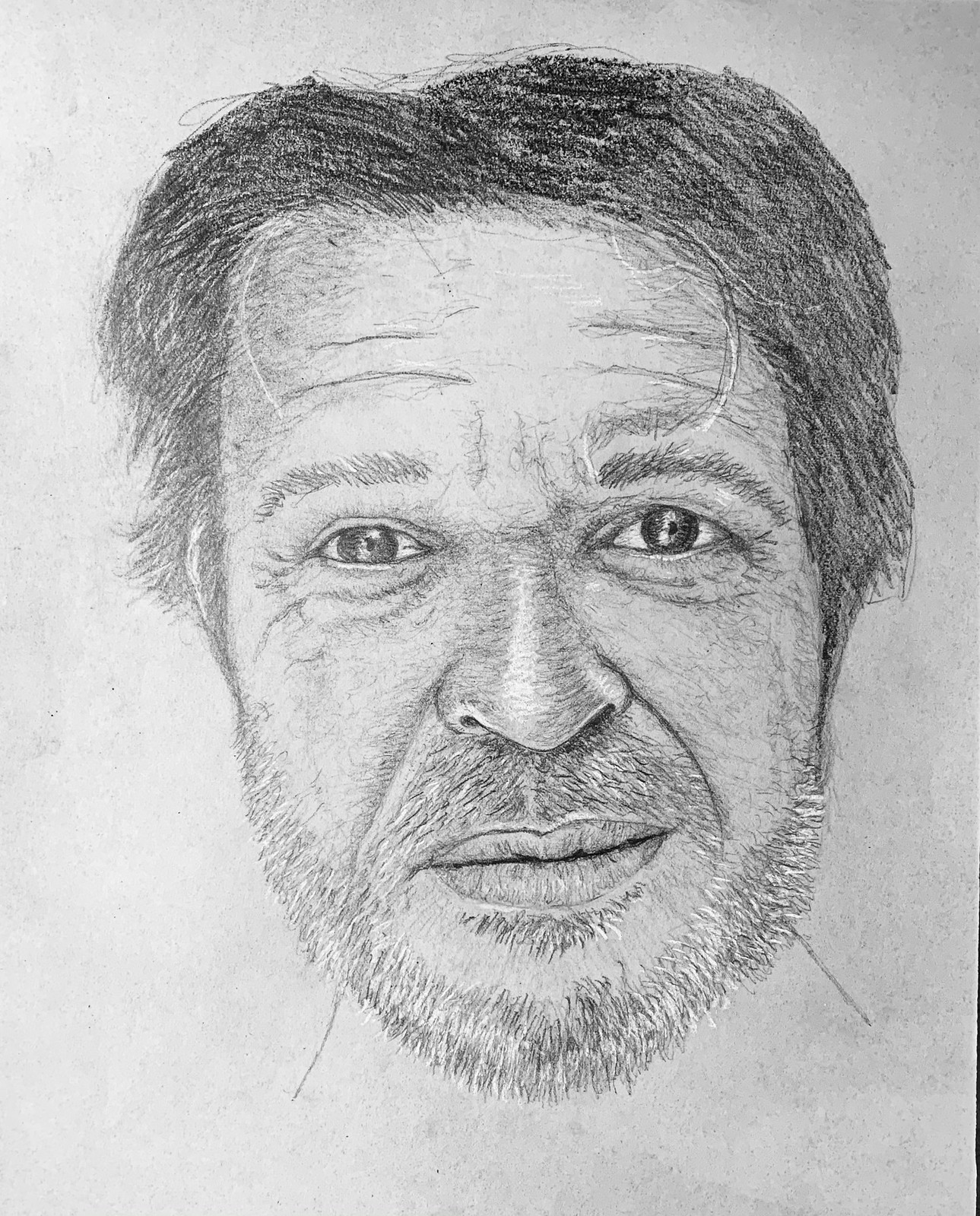This image is a highly detailed black and white pencil sketch of a middle-aged Caucasian man. The man has a light beard, indicative of several days of growth, which extends partially to his mustache and chin. His hair, parted slightly off-center, appears somewhat disheveled, with strands hanging over his eyebrows and longer sections falling just above his ears. The weathered, serious expression on his face is accentuated by distinct forehead lines and dark, tired-looking eyes. The left eye is more open and typically shaped, whereas the right eye appears a bit lazier, adding to the somber tone. Shading adds depth to his prominent nose and subtly marks what would be the start of a neck. The background is a stark white, emphasizing the intricate, sketchy details of his face and hair. The overall impression is of a weary, perhaps sad, man captured in a raw, realistic manner.